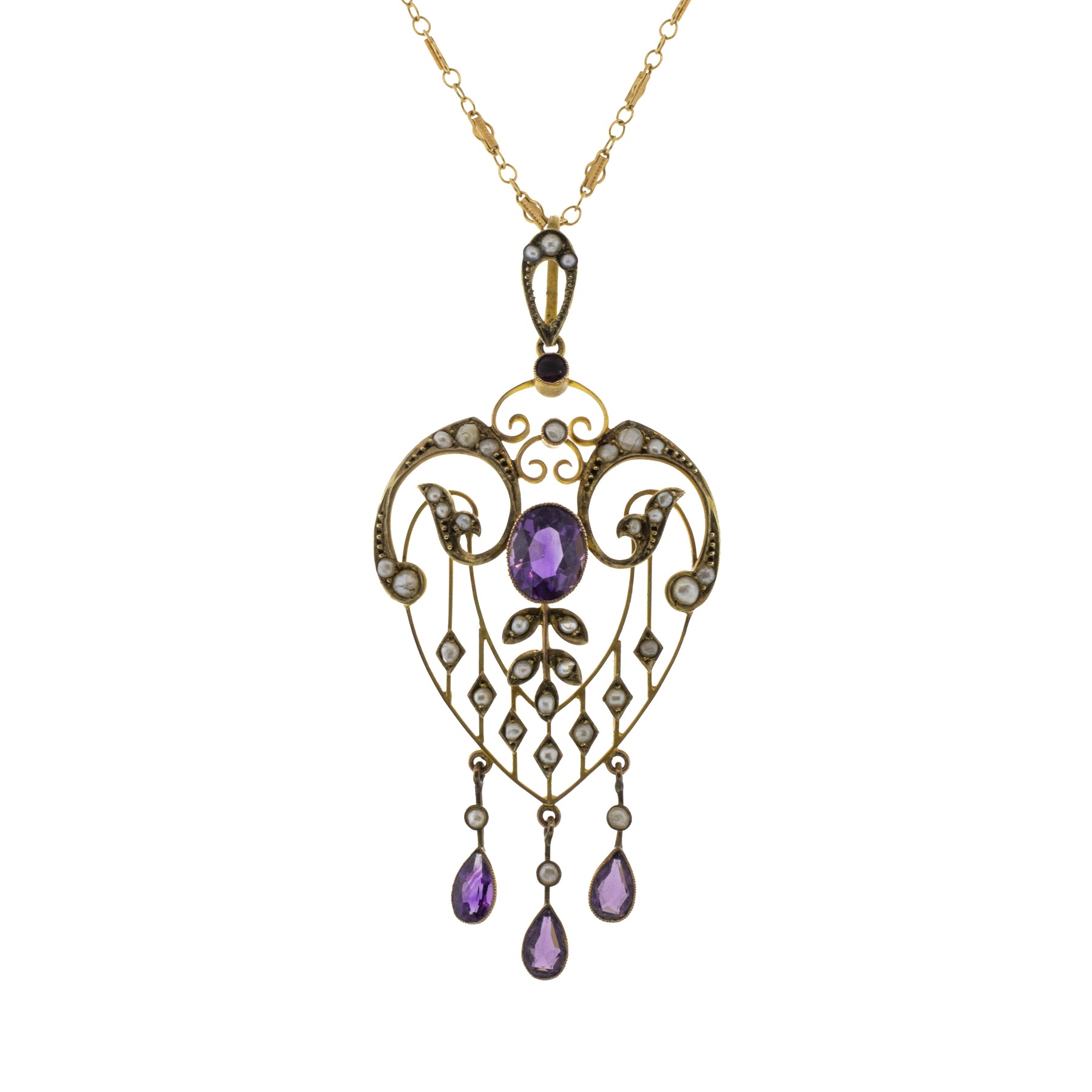A full-color, vertically rectangular photograph against a white background showcases a meticulously designed necklace. The gold chain features interconnected circular links and attaches to a shield-shaped black section, adorned with three white stones. Central to the necklace's design is an ornate golden heart-shaped fixture, with elegant swirls extending to the left and right, each embedded with additional white stones. At the center of this heart-shaped design lies a prominent purple gemstone. From its bottom, three teardrop-shaped purple gemstones gracefully hang. The overall display captures the intricate blend of gold, black, and purple elements, highlighting the detailed craftsmanship of the piece.